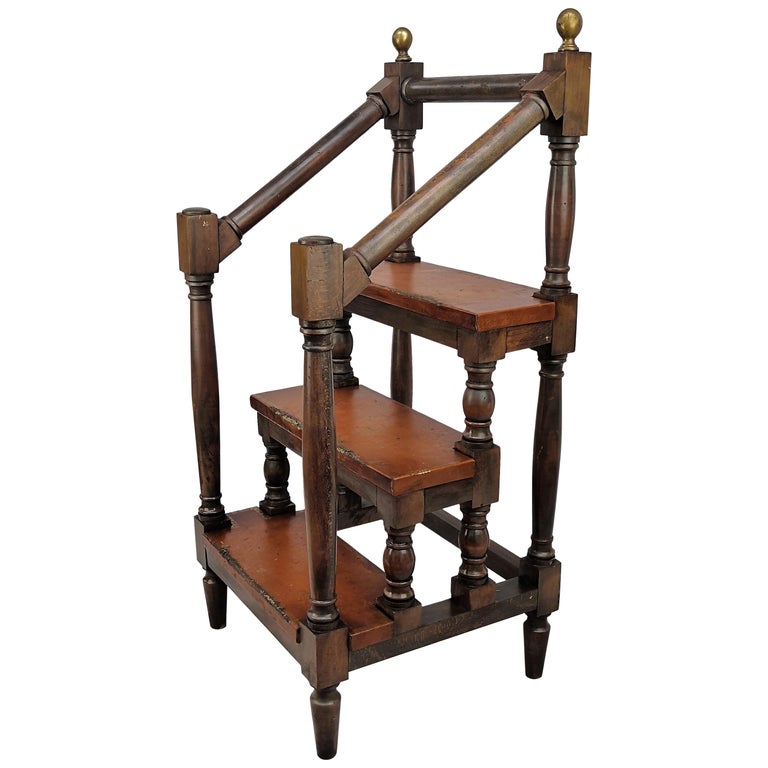This image showcases an antique wooden step stool with three well-worn steps. The frame and railings are crafted from dark wood, likely oak, while the steps themselves are a lighter, reddish oak tone, reflecting significant use. The stool features smooth, carved railings with brass knobs positioned at the top by the third step, adding a touch of elegance. The knobs are slightly oval-shaped, contributing to the antique aesthetic. The stool is designed to be portable, standing on four legs that resemble those of an old-fashioned coffee or kitchen table. With its combination of dark and lighter wood tones, this functional piece is ideal for use in libraries or kitchens to reach high shelves and cabinets.